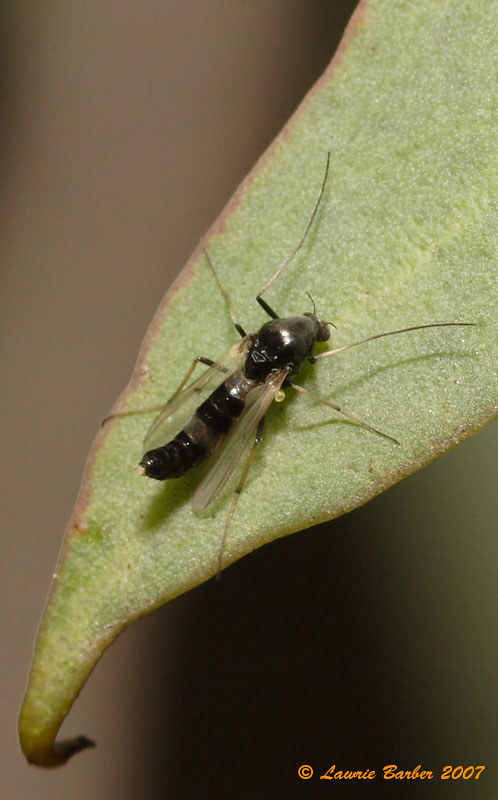This detailed close-up photograph captures a striking insect perched delicately on the tip of a green leaf with reddish edges. The insect, black with silver stripes patterned along its body in alternating sections, showcases a distinctive appearance with its transparent wings and six long, thin legs, two of which are notably extended towards the front. The head of the insect appears small compared to its body, which reveals in closer inspection to be predominantly its back. The photo, expertly taken by Lori Barber in 2007, isolates the insect as the central subject by blurring out the background, ensuring that the viewer's entire focus is on the intricate details of the bug. The image is in portrait orientation and features the photographer's copyright information at the bottom right, written in orange script.